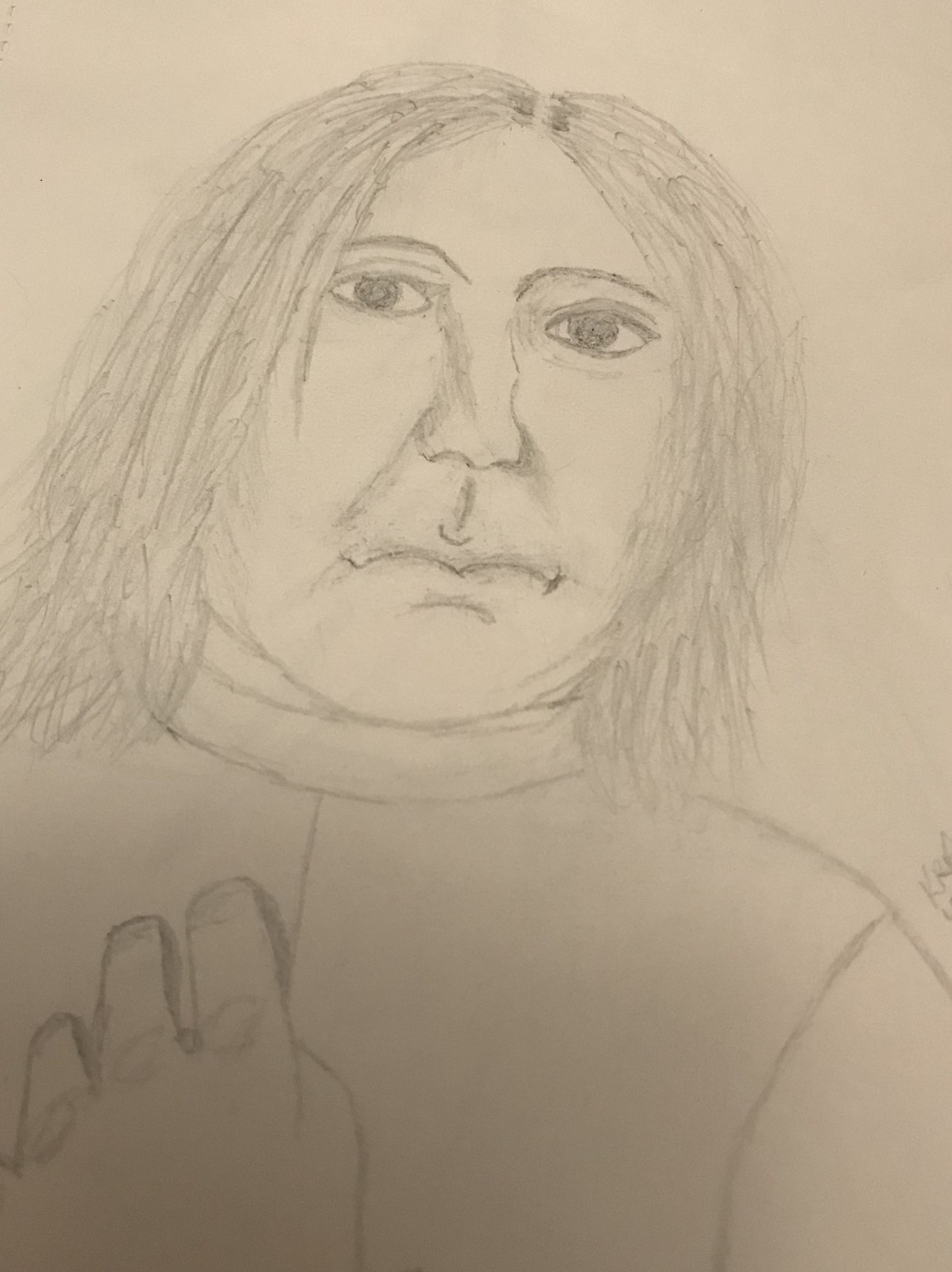A detailed close-up image of a pencil drawing on white paper. The drawing focuses on a person whose head tilts slightly to the right. The individual's head is oval-shaped with hair that mostly brushes their shoulders, but features distinctive side bangs in the front. The person's face includes detailed, oval eyes with a dark pupil and a white highlight on the left side of each eye. Noticeably sharp eyebrows and a pronounced, pointy nose also characterize the face. The person is depicted wearing a shirt that conceals part of their neck, and one hand is visible in the frame, though only three fingers are drawn. The extreme zoom of the image excludes any view of the paper's background or what it rests upon.